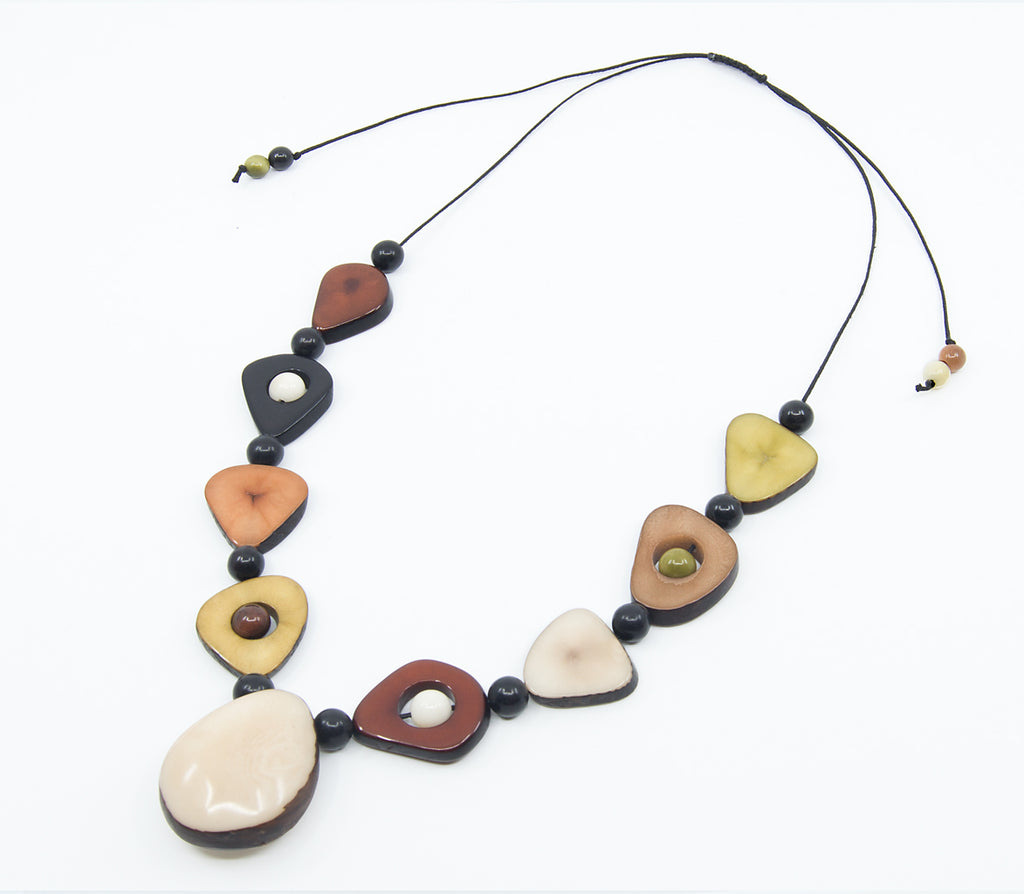This is an image of a necklace, lying flat against a white background, possibly a table or piece of paper. The necklace is held together by black string, which arches at the top right of the frame. An additional arch of black string, attached to two beads on either side - a green and black bead on the left and a brown and white bead on the right - is also visible. The main portion of the necklace features a series of alternating black beads and triangular-shaped pieces with rounded corners, arranged in a counterclockwise pattern. 

Starting from the bottom left and moving upwards, the sequence includes: a dark brown triangular piece, a black triangular piece with a white bead in the center, a light brown triangular piece, a very pale green triangular piece, a large white triangular piece at the bottom tip of the necklace, a reddish-brown triangular piece with a white bead in the middle, another white triangular piece, and a light brown triangular piece with a green bead in the middle. The pattern culminates with another very pale green triangular piece, each side bracketed by a black bead, producing an intricate and colorful design with hues of yellow, white, reddish brown, green, and black interspersed throughout. The black string is wound tightly at the top, ensuring the necklace's delicate yet vibrant components are securely connected.